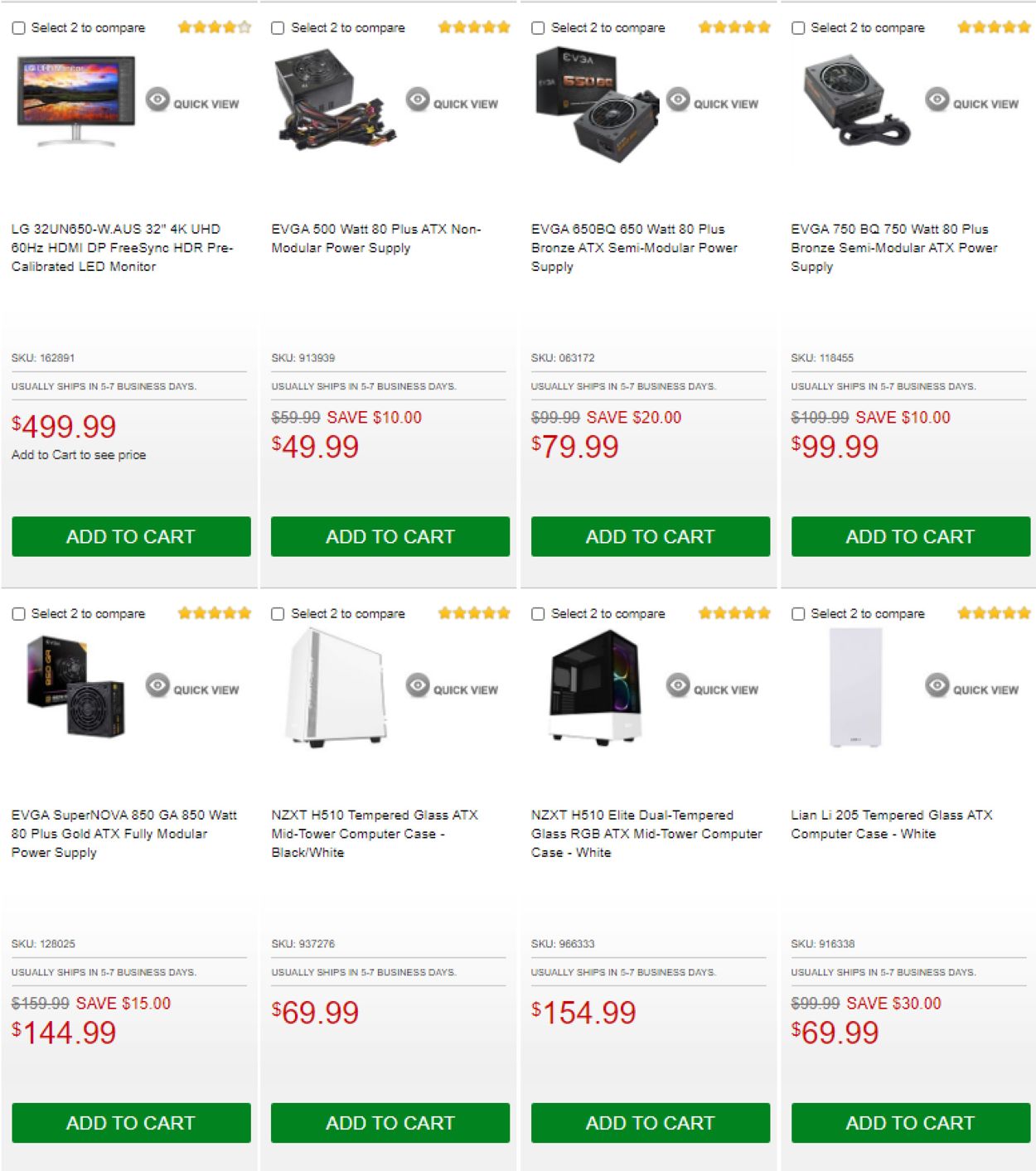This screenshot depicts a webpage showcasing a variety of computer-related items, each presented against a clean, white background. The first item on the top row is an LG 32-inch 4K UHD LED monitor, with features including a 60Hz refresh rate, HDMI and DP ports, FreeSync technology, HDR support, and pre-calibrated settings. This monitor is listed at a price of $499, highlighted in red text, with an instruction in black text to add the item to the cart to see the final price. It has received a rating of 4 out of 5 stars.

Next to the monitor, there is an EVGA 500W 80PLUS ATX non-modular power supply priced at $59.99, but currently available for $49.99 after a $10 discount (displayed in red text). This item has a perfect rating of 5 out of 5 stars. Adjacent to this is the EVGA 650VQ 650W 80PLUS Bronze ATX semi-modular power supply, originally priced at $99.99. After a $20 discount, it is listed at $79.99, also rated 5 out of 5 stars. The final item in this row is the EVGA 750VQ 750W 80PLUS Bronze semi-modular ATX power supply, reduced from $109.99 to $99.99 after a $10 discount, maintaining a rating of 5 out of 5 stars.

In the second row, the first item is the EVGA Supernova 850GA 850W 80PLUS Gold ATX fully modular power supply. Initially priced at $159.99, it is now $144.99 after a $15 discount, though it lacks a visible rating. Next is the NZXT H510 tempered glass ATX mid-tower computer case available in black and white, priced in red text at $69.99. Following this, we have another case, the NZXT H510 Elite Dual Tempered Glass RGB ATX mid-tower computer case in white, with a red price tag of $154.99. Finally, there is the LIAN 205 Tempered Glass ATX computer case in white, originally priced at $99.99 but currently available for $69.99 after a $30 discount.

All items feature an "Add to Cart" button in green with white text for user convenience.